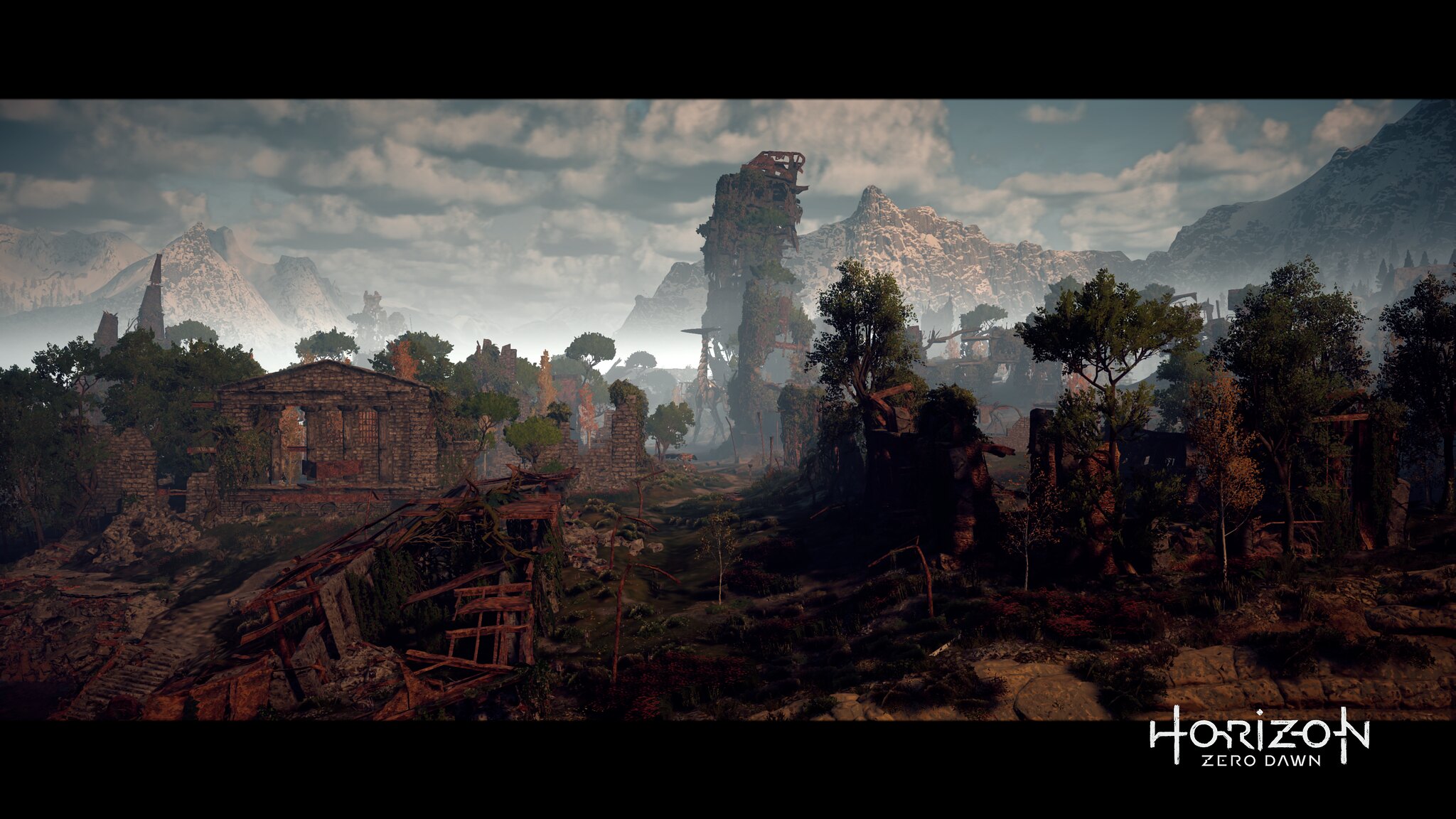The image is a highly detailed, computer-generated scene from the video game "Horizon Zero Dawn," with the game logo prominently displayed in white text at the bottom right corner. The landscape features a ruined, apocalyptic setting with a diverse range of environmental elements. Dominating the background, majestic snow-capped gray mountains stretch across the scene under a blue sky filled with fluffy clouds. In the midground, towering, slender trees with green leaves stand amid the devastation. The scene depicts numerous crumbling and abandoned buildings, some constructed from stone with visible pillars, while others are dilapidated wooden and rusty metal structures scattered and collapsed across the desolate ground. Brown debris and stones litter the foreground, adding to the chaotic and war-torn ambiance. The overall image conveys a dramatic and immersive post-apocalyptic world, emphasizing the contrast between natural beauty and man-made destruction.